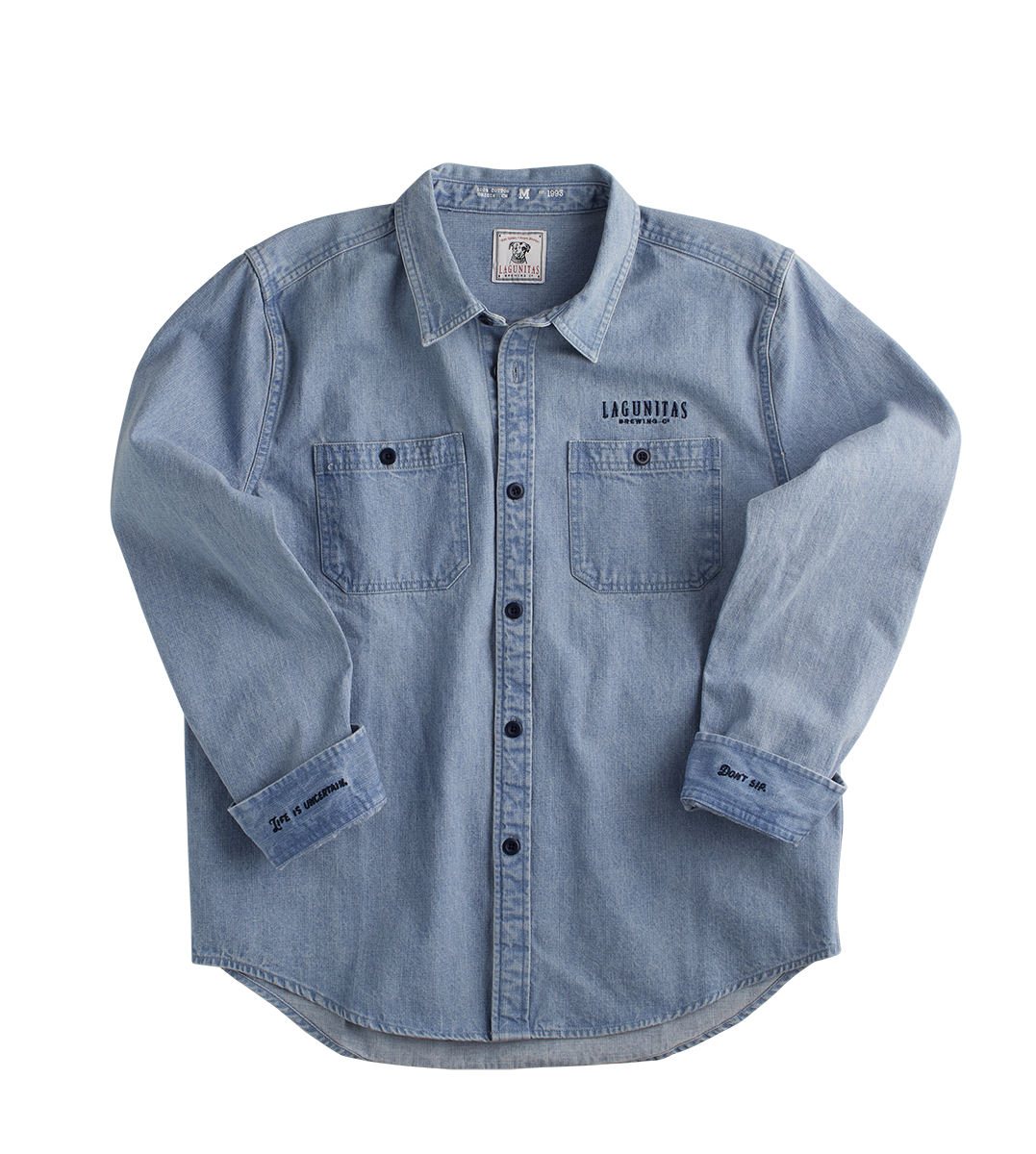The image showcases a light baby blue denim jacket, commonly used as a stock photo for apparel. The jacket features two chest pockets, each secured with buttons. Above the right pocket, the word "Lagunitas" is written, indicating branding associated with Lagunitas Brewing Company. A white tag inside the collar also bears the "Lagunitas" name and depicts a dog with floppy ears. The jacket is a size medium, as denoted by the "M" above the dog logo on the tag.

The jacket's design includes black buttons running down the middle. Intricate details include embroidery on the cuffs; the right cuff reads "Life is Uncertain," while the left cuff states "Don't Sip." The cuffs are rolled up slightly to better display this embroidery. The overall cut of the jacket tapers slightly upwards toward the hips, adding to its stylish appearance.